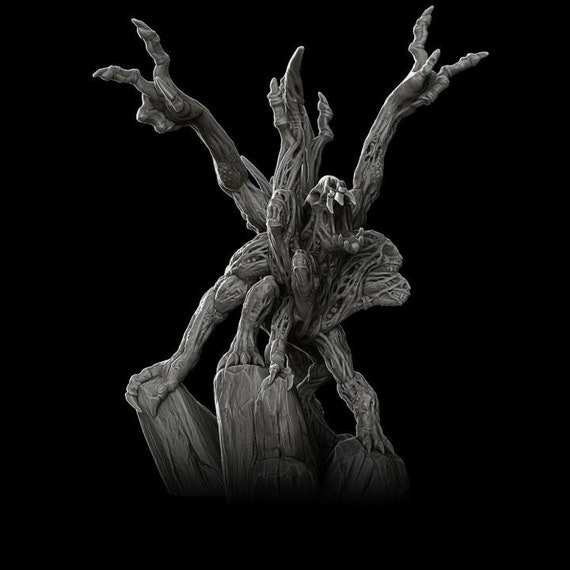A computer-rendered 3D fantasy figure is depicted against a solid black background. Illuminated by a light source from the upper left, the gray-hued beast's edges are strikingly highlighted. The creature stands on four legs, each ending in long, sharp claws. Its body, reminiscent of a twisted, tree-like form, converges at the center where four extended arms, each with three clawed fingers, protrude menacingly. The beast's face features a small skull with pronounced openings for eyes and ears. Its wide-open mouth reveals rows of long, white teeth, giving the impression of a powerful roar. The figure stands on three rocky structures, which seamlessly blend into the black background towards the bottom of the image.